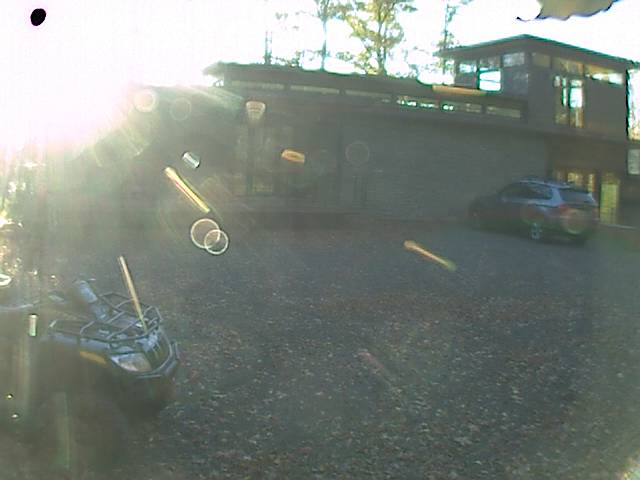This image captures a blurred photograph of a very modern-looking house under bright sunshine that obscures the left side of the image with glare. The modern house predominantly features gray brick and a flat black roof, with a distinctive two-story section on the right side. The building also boasts large windows on the upper story, some of which appear to encircle the top like a turret. The left side of the image showcases the front half of a shiny black car, while a shiny SUV or possibly an ATV, which gives an impression of having a mini cage or a distinctive hood ornament, is parked directly in front of the house pointing towards it. The entire foreground consists of bare earth or a black asphalt parking lot.